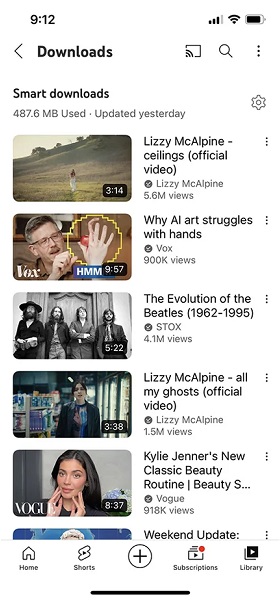This image depicts the screen of a device with various icons and text. In the top left corner, the time is displayed as 9:12. Moving to the top right corner, there is a cellular signal icon, followed by a Wi-Fi icon, and finally a battery icon indicating the device's battery status. Below this, a black left arrow points to the left, accompanied by the text "Downloads."

Further down, the screen shows the section titled "Smart Downloads," noting that 487.6 MB has been used, and the last update was completed yesterday. To the right of this information is a settings icon. Underneath, the content reads "Izzy McPine - Ceilings (Official Video)," though there seems to be a slight misspelling in the artist's name, which should be "Lizzy McAlpine." It indicates that the video has 5.67 views, suggesting either an error or missing context.

Below this, there is another entry titled "YAI Art Struggles With Hands," followed by the channel name "Vox," which has accumulated 900K views.